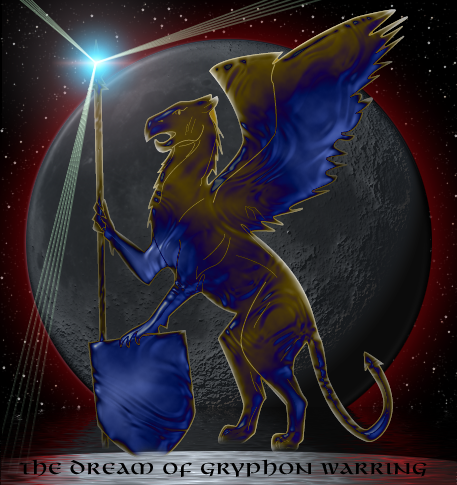This image is a detailed piece of digital art set against a white-to-red gradient background, featuring an intricate science fiction theme. Dominating the scene is a majestic Gryphon, portrayed standing upright on its hind legs with a pair of grand eagle wings extending from its back and a long, pointed tail. The Gryphon's body showcases a vibrant swirl of blue and yellow patterns that mix into different shades across its form. Its left hand props a shield against the ground, while its right hand brandishes a large spear. The spear's tip emits a radiant white light, creating streaks that spread across the image. Positioned behind the Gryphon is a glowing moon with a red halo, set against a star-studded night sky that enhances the otherworldly ambiance. At the bottom, the text "The Dream of Gryphon Warring" is written in an old-style font, grounding the fantastical imagery with an evocative title.